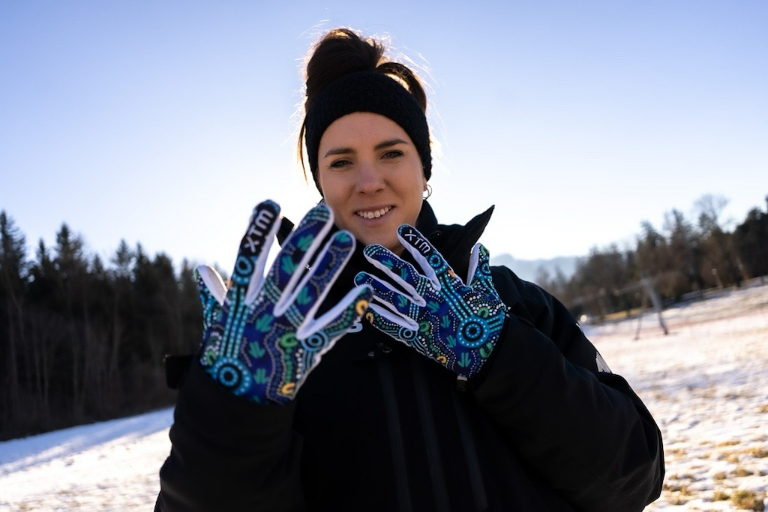In this outdoor daytime photograph, a smiling woman is centrally framed from the waist up against a blurred backdrop of a blue and white sky and pine trees. Beyond the trees, distant mountains are faintly visible. The woman, of Caucasian descent with light skin and straight brown hair pulled into a messy ponytail, adorns a large black headband covering part of her forehead. She is dressed in a long-sleeve, puffy black coat. Her arms are bent, with both hands open and fingers spread, showcasing gloves that are white on the palm side and adorned with blue and green patterns resembling beadwork on the back. The ground is snow-covered, with scattered small bushes and leaves adding texture to the scene.